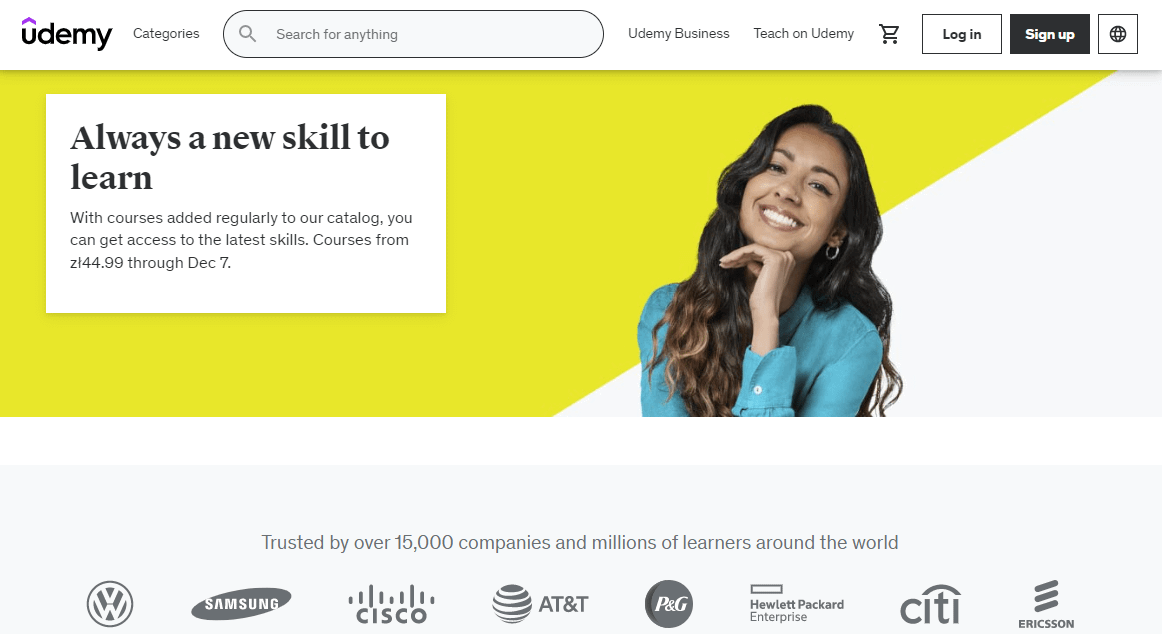The image is a screenshot from the Udemy website or app, showcasing a wide, rectangular banner that is about twice as wide as it is tall. At the top of the image, the Udemy logo is prominently displayed, featuring the name "Udemy" written in black text with a medium purple up-arrow accent over the 'U'. To the right of the logo are various navigational options: "Categories," a search bar, "Udemy Business," "Teach on Udemy," a shopping cart icon, "Login" button, "Sign In" button, and a globe icon. 

The main banner below this toolbar has a predominantly yellow background with a diagonal white section occupying the lower right corner, roughly covering 25-30% of the banner. Inside this white space, towards the right, there is an image of a woman smiling warmly with long, wavy dark brown hair resting her head on her hand.

On the left side of the banner, there is a text box with a white background. Large, bold black lettering reads, "Always a new skill to learn," and beneath it, smaller text states, "With courses added regularly to our catalog you can get access to the latest skills courses from $4.99 through December 7th."